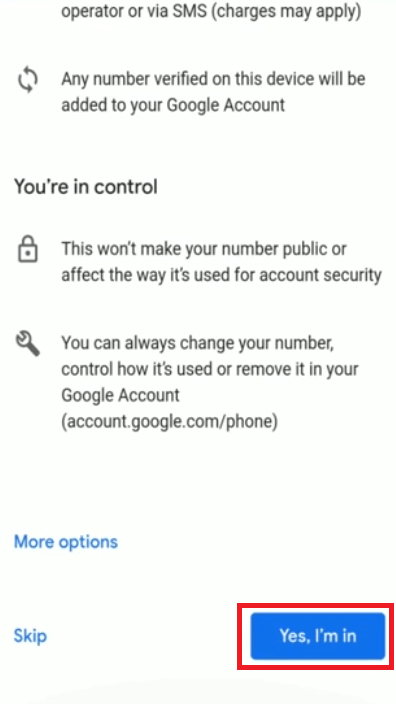The image is a screenshot of a user interface within an application, guiding users through the process of linking a phone number to their Google account. At the top, on a white background with gray text, it reads, "Operator or via SMS, charges may apply." Below this text are two circular arrows, signifying a process or ongoing action.

In the main body of the screenshot, there's a section emphasizing user control over their number with the message, " This is any number verified on this device will be added to your Google account. You're in control." Accompanying this message is a lock icon, reinforcing security and privacy. It clarifies that adding a number "won't make your number public or affect the way it's used for account security."

Further down, an image of a gray wrench represents settings and customization. The text indicates, "You can always change your number, control how it's used, or remove it in your Google account," and provides the URL "account.google.com/phone" for additional management.

Towards the bottom of the interface, there’s a blue hyperlink for "More options," and a “Skip” option also highlighted in blue, placed to the left.

Finally, a prominent red rectangular box highlights a blue button that says, "Yes, I'm in," which is meant for users to confirm their agreement to link the phone number to their account.